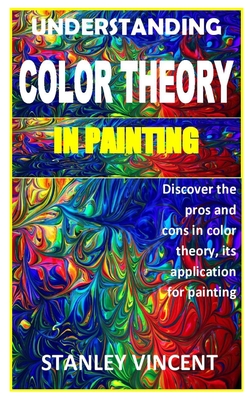The image depicts a vibrant book cover with an intricate interplay of colors resembling stained glass or a watercolor painting. Predominantly featuring reds, blues, greens, yellows, and some purplish hues, the background showcases multiple rectangles where the colors blend at the edges while maintaining distinct borders. Positioned at the very top in bold white text is the title "Understanding Color Theory," followed by "In Painting" in a vivid yellow. Towards the bottom right of the cover, the text reads, "Discover the Pros and Cons in Color Theory, Its Application for Painting," underscoring a detailed exploration of the subject. The book is authored by Stanley Vincent, with his name clearly displayed in white at the bottom. The entire cover is framed by a thin yellow outline, adding a coherent structure to the colorful, swirl-like patterns within.